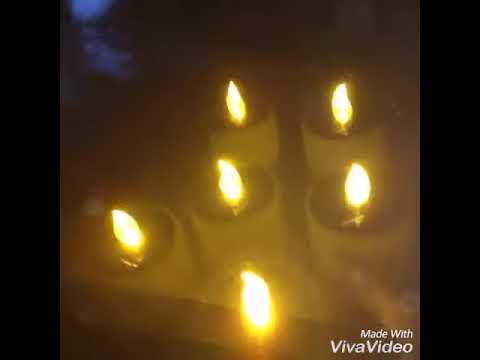The indoor photograph captures an overhead view of a series of six electric light candles arranged in a distinct pattern. The candles are configured with two on the left, three on the right, and one in the center, creating a layout that suggests a partial circle missing one candle at the top. The black candles are held in white holders, and each emits a yellow flame, casting a warm gold-amber glow. Framing the scene are two large black and white rectangular panels on either side, each occupying around 20% of the photo. At the bottom-right corner, the image is marked with the text "Made with Viva Video."